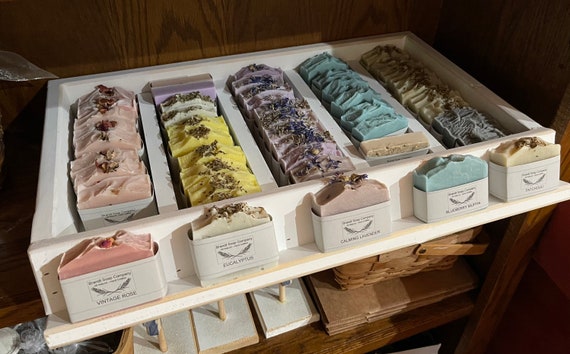The image depicts a white wooden storage drawer with five compartments, nestled against a dark brown pine wood wall. Each compartment contains a row of square soap packages, thoughtfully arranged and lined with color-coded tissue paper in soft pastel shades: pink, yellow, lilac, blue, and a creamy off-white. The soaps are attractively packaged and appear to be potential gifts or party favors, such as those for a baby shower or wedding.

The first row of soaps, on the far left, is pink and labeled "Vintage Rose." Behind this soap is a line of identical pink soaps. To the right, the second row features yellow soaps labeled "Eucalyptus," followed by a row of purple soaps named "Calming Lavender." The blue soaps in the fourth compartment are difficult to read but might be "Blueberry," and the final row of creamy-colored soaps could be labeled "Patchouli," although the label is not clear. 

These soaps are arranged on a shelf with additional items, including a basket and various boxes, placed on a second lower shelf, contributing to a cozy and well-organized display. The overall aesthetic suggests a setting in a boutique or a specialized store, offering an appealing and orderly presentation of handcrafted soap products.